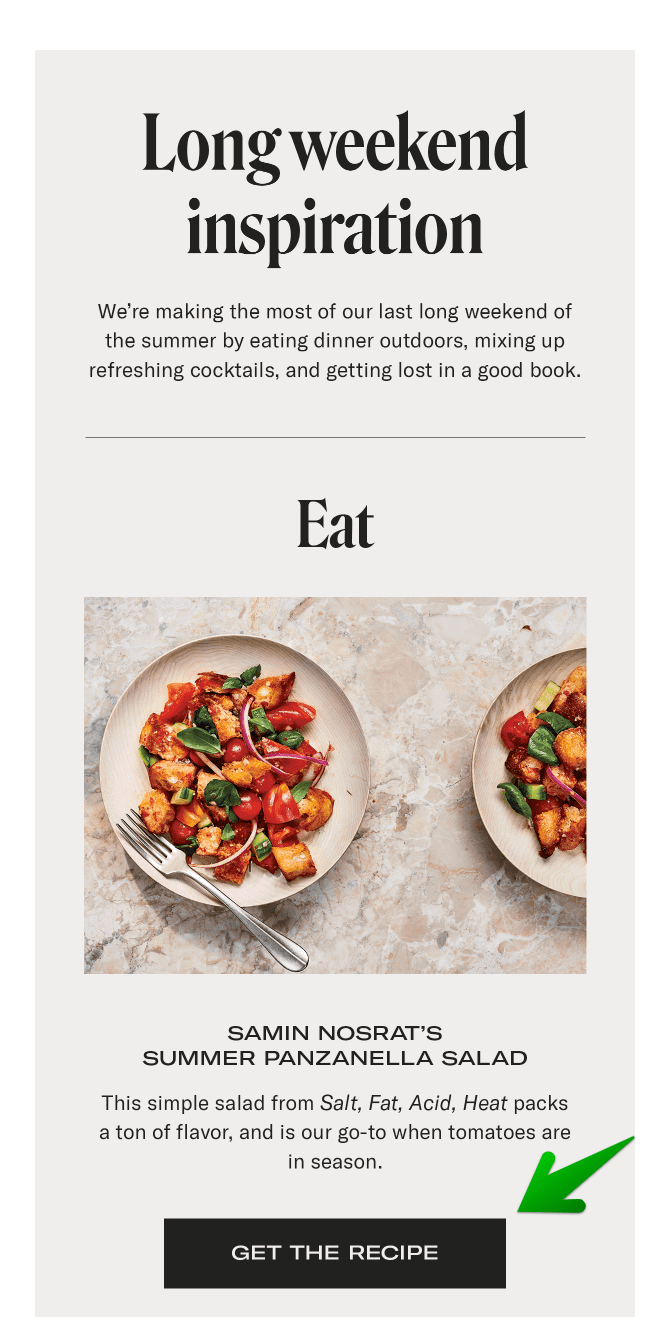This image features a cropped section of a recipe website. The background is a clean white, providing a crisp and uncluttered look. At the top of the page, bold text reads "Long Weekend Inspiration," followed by a subheading that states, "We're making the most of our last long weekend of the summer by eating dinner outdoors, mixing up refreshing cocktails, and getting lost in a good book." Beneath this, the section is titled "Eat," showcasing a vibrant photograph of a dish served on plates, with a fork placed to the left. The plates rest on an elegantly patterned surface featuring shades of brown, white, and black. Below the image, text introduces "Samin Nosrat's Summer Panzanella Salad," highlighting it as a simple yet flavorful option perfect for when tomatoes are in season. A prominent black button with white text reads "Get Recipe," accompanied by a green arrow pointing towards it, guiding users to the recipe link.